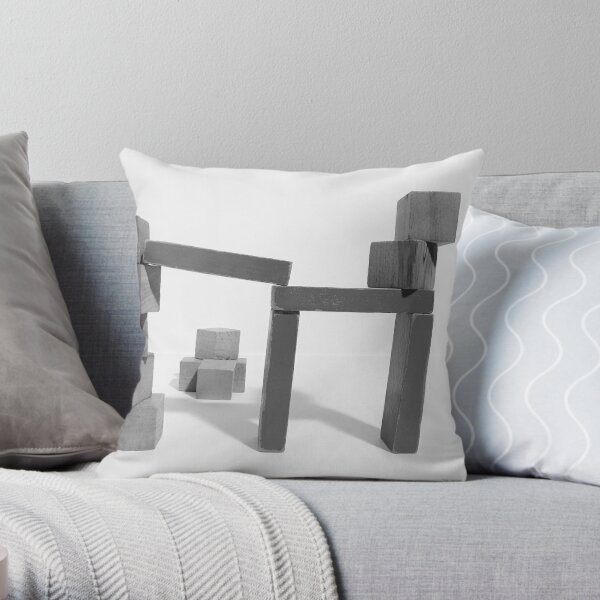The photograph features a close-up of a light gray sofa adorned with various pillows and a blanket, set against a light gray wall. Dominating the center of the frame is a uniquely designed white pillow showcasing an intricate black and white print of stacked wood blocks, creating structures reminiscent of Stonehenge with a mix of tall, skinny blocks and thicker ones, some of which lie in small piles on the ground. On the left side of the sofa, partially visible, is a large gray pillow accompanied by a very light gray woven blanket that drapes over the corner. To the right, there is a light gray pillow decorated with wavy white lines. The overall color palette of the scene is muted, featuring shades of gray, white, and silver.